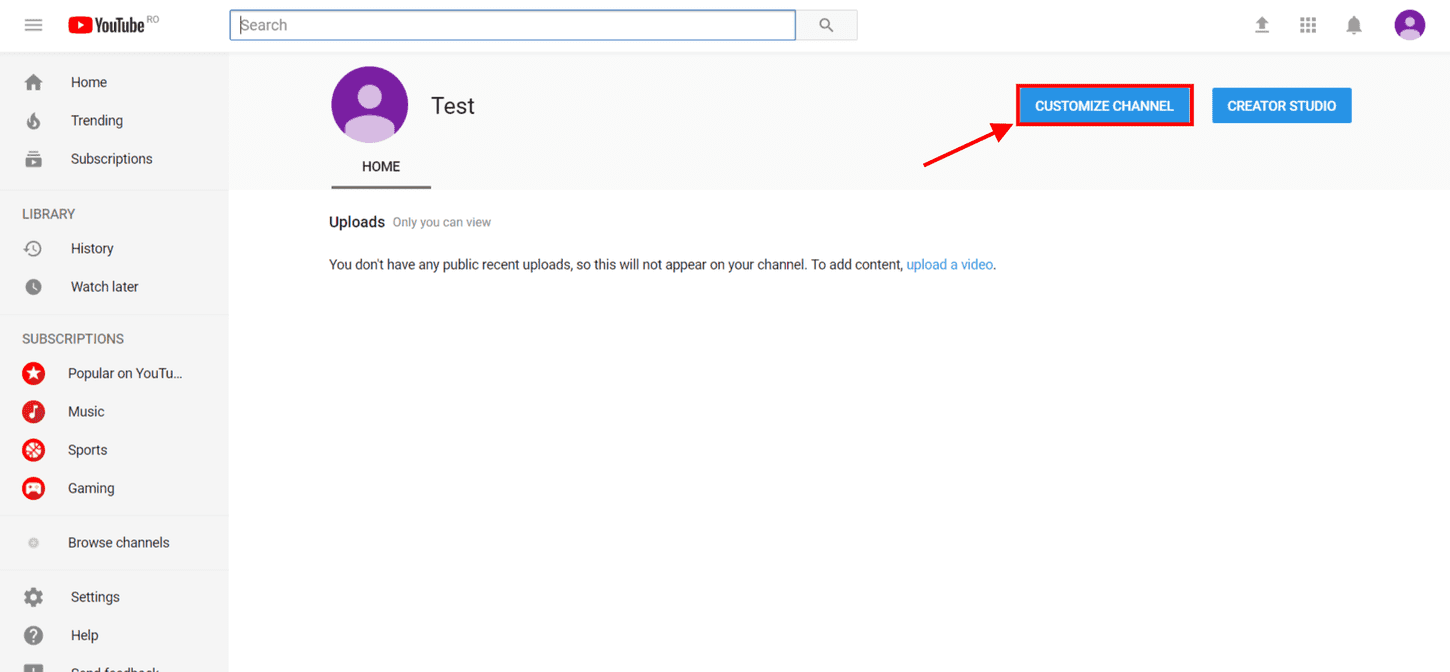This image captures the user interface of a YouTube webpage. Dominating the top left corner is the iconic YouTube logo, a red box with the word "YouTube" in black text. Adjacent to the logo are three horizontal gray bars, indicative of the menu icon. 

At the top of the page lies a search bar accompanied by a search icon. Moving rightward, there is an arrow with an underline, designated for downloading. Nearby are a box with dots representing additional options, an alert icon, and a purple person icon signifying the user profile.

The main body of the website features a prominent gray bar stretching across the screen. Displayed on this bar are the labels, including "Test" and "Home." Situated on the right side of the bar is the "Customize channel" button outlined in blue with a red perimeter, along with the "Creator Studio" button highlighted in blue. A red arrow points towards the "Customize channel" button.

Beneath the "Home" label, it indicates, "Uploads - only you can view." Following this is a disclaimer stating, "You don't have any public recent uploads so this will not appear on your channel," and prompts the user to "Upload a video." The phrase "Upload a video" is emphasized in blue.

On the left panel, a gray box lists various sections such as "Home," "Trending," and "Subscriptions." Under the "Library" section, items listed include "History," and "Watch later." In the "Subscriptions" section, noteworthy categories such as "Popular on YouTube," "Music," "Sports," and "Gaming" are displayed. At the bottom, options labeled "Browse channels," "Settings," and "Help" appear, though the last item is partially cut off.

The layout and details provide a comprehensive glimpse into the user's YouTube channel interface, richly populated with navigational and functional elements awaiting interaction.